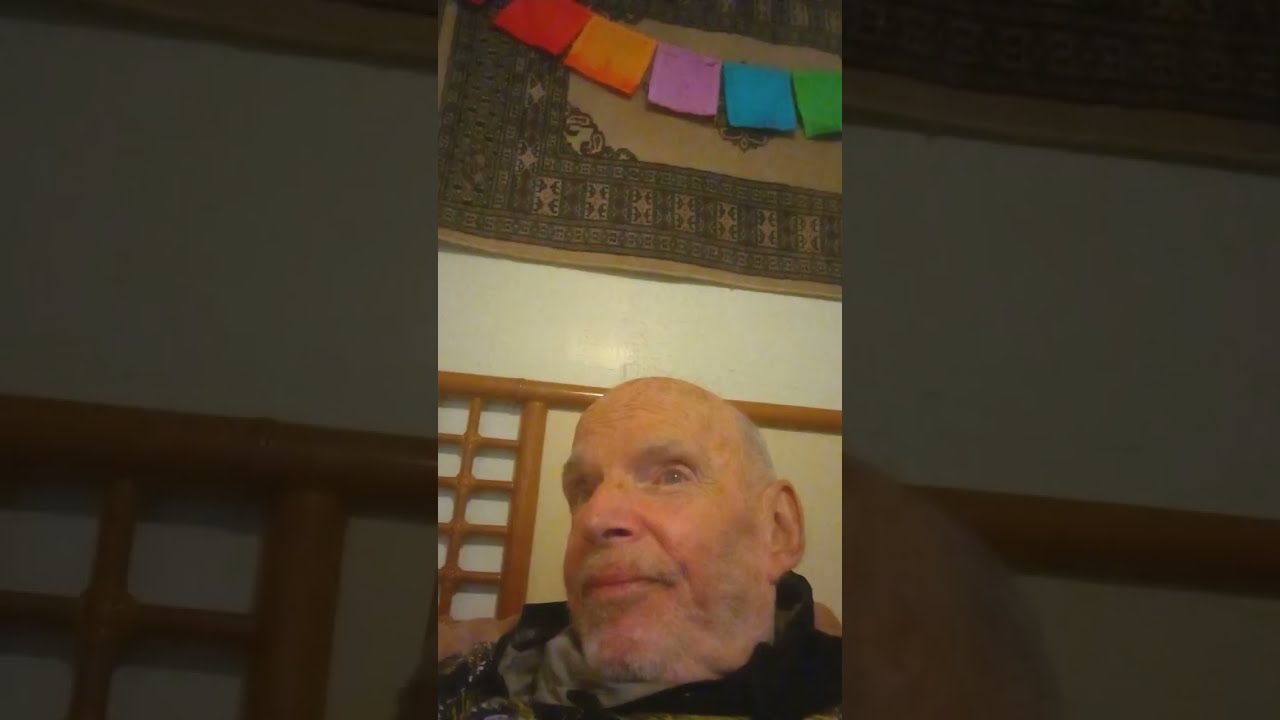This photograph features an older Caucasian man with a bald head, except for a few gray hairs above his ears, and a scruffy beginning of a white beard. He is visible from the shoulders up and is centered in the image, looking slightly to the left. He wears a dark or black shirt. The background comprises a detailed tapestry with a light brown center and dark brown designs, possibly depicting buildings or blocks. Draped across the middle of this tapestry is a colorful banner featuring squares in red, orange, purple, blue, and green, arranged in a curved line. The setting appears to be indoors, in a room with elements that might suggest an Asian influence, such as the decoration on the wall behind him. There are also wooden bars visible in the background and brown trim on the wall. Lighting in the image is artificial, likely provided by a ceiling fixture, giving the overall scene a clean yet slightly dim ambiance. The photograph might depict a picture within a picture format, as the corners of the image exhibit a dark gray overlay, providing a sort of zoomed-in effect on the man's face and the textured, beige wall behind him.